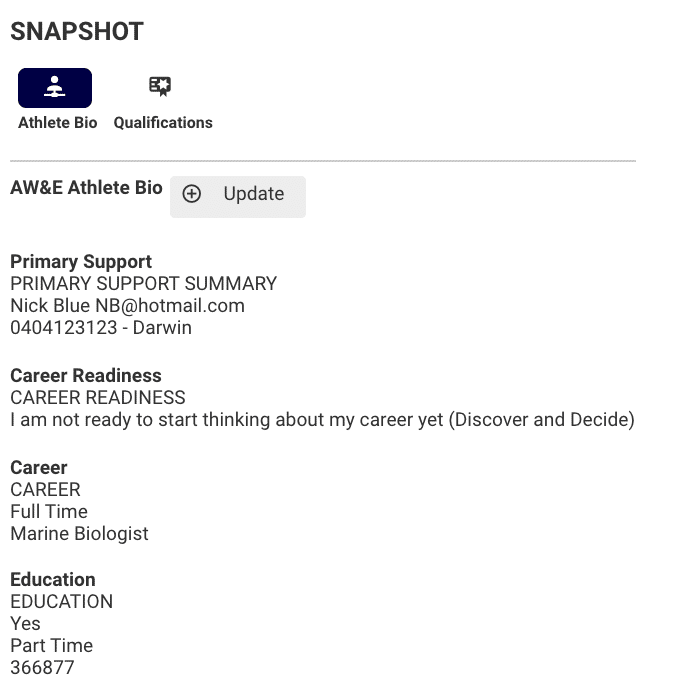This image appears to be a screenshot of an athlete's online profile or resume on a website. The page is titled "Snapshot" and features two main sections: "Athlete Bio" and "Qualifications." The "Athlete Bio" section is highlighted with a dark blue color, indicating it is currently selected. An icon of a person is next to this section, whereas the "Qualifications" section, represented by a gold ribbon icon, is empty.

Beneath these sections, the header "W&E Athlete Bio" is displayed. Adjacent to it, there is a clickable button labeled "Update" with a plus sign. Below this, the primary support contact information is listed as Nick Blue, with the email address "nick.blue@hotmail.com" and phone number "0404-123-123" affiliated with Darwin.

The profile includes various sections providing insights into the individual's career readiness, goals, and contact details. Under "Career Readiness," the entry reads, "I am not ready to start thinking about my career yet." However, the section labeled "Discover and Decide" states "Career: Full-time marine biologist." The "Education" category is noted with "Yes, part-time." Additionally, numbers such as "366877" are listed, whose specific significance is unclear.

The page background is white with black text, providing a clean and simple layout. A small horizontal line separates the "Athlete Bio/Qualifications" header from the "W&E Athlete Bio," suggesting a structured format. Overall, the content seems to resemble a preliminary or incomplete athlete's resume with placeholder sections for further details.